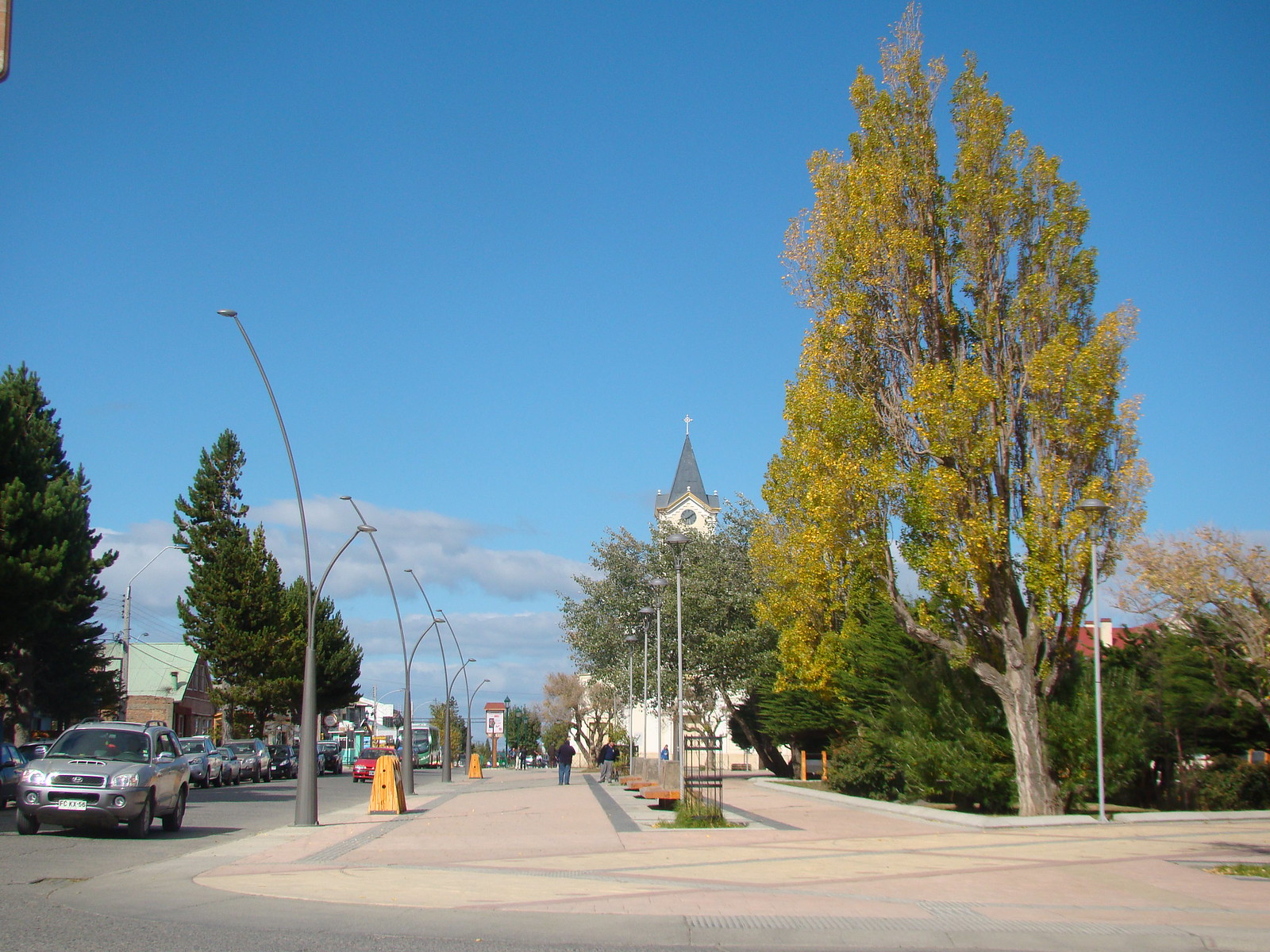This color photograph captures a vibrant small-town street scene bathed in sunlight and marked by clear blue skies with just a few clouds in the distant background. Running down the center of the image is a road lined with parallel-parked cars on the left side, while a couple of vehicles are seen driving further down the street. On the right side of the road stands a series of double-sided street lamps; these feature tall fixtures arching over the road, partnered with shorter lamps arching over the adjacent sidewalk. There are at least four of these prominent lamp posts fading into the background.

The sidewalk itself, smooth and fairly flat, is dotted with a few pedestrians either walking or engaged in conversation. On the left side of the image and lining the street is a row of tall trees, some of them blooming with small yellow flowers, contrasting with a mix of green foliage and a couple of pine trees. Further to the right, behind another sidewalk, lies a small park area filled with lush green bushes and various shrubbery. In the distant background, the steeple of a church punctuates the skyline, adding a quaint architectural element to the scene. The overall atmosphere is calm and serene, highlighting the charming nature of the town without any identifiable landmarks to hint at its specific location or the year.